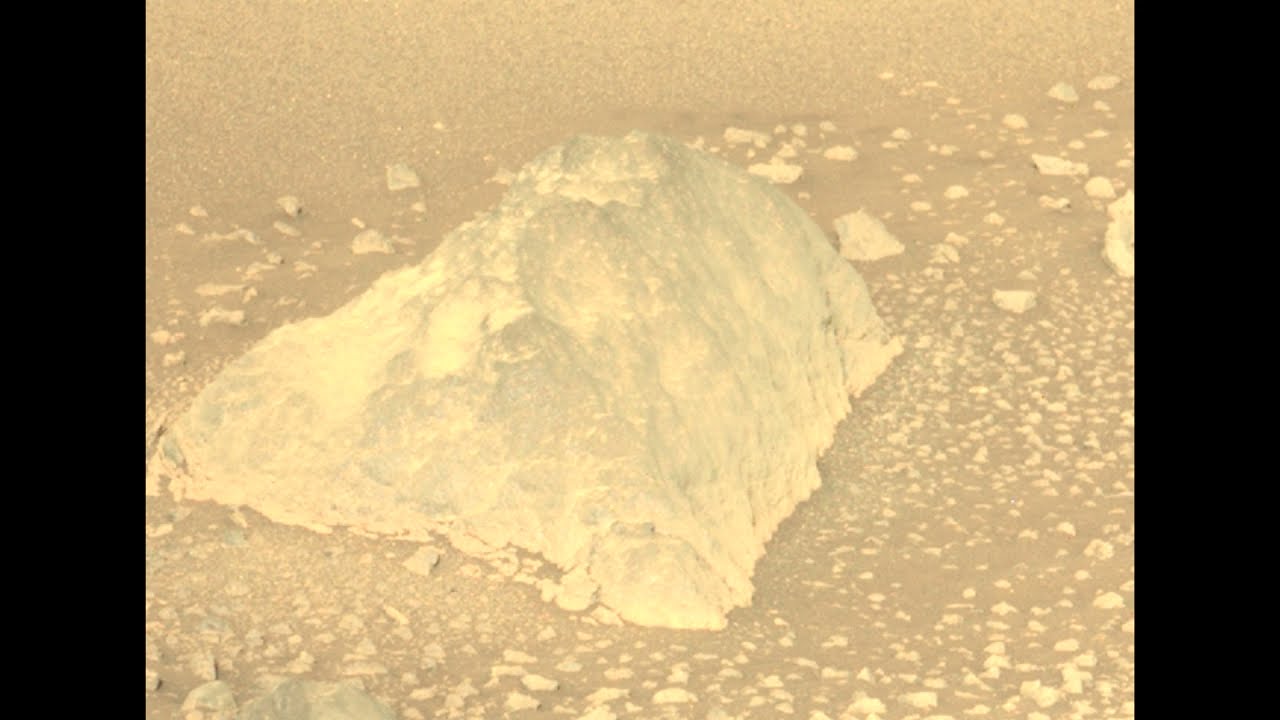The horizontal rectangular image features vertical black borders on either side, creating a near-square shape in the center. Dominated by a rugged and desolate landscape with sepia-like tones, the image portrays a large, beige rock formation or cliff at the center. This central structure appears to be surrounded by numerous scattered stones and broken rock fragments, giving an impression of a weathered and eroded terrain. The top section of the rock formation is smoother and more intact, while the middle and lower sections are strewn with both large chunks and smaller consistent pieces. The background remains consistent with the earthy, off-yellowish hues, devoid of any discernible text, adding to the barren and somewhat eerie atmosphere. The overall scene could resemble a distorted or filtered view, possibly as if taken from a sonar or video screenshot, emphasizing the rough and fragmented nature of the landscape.